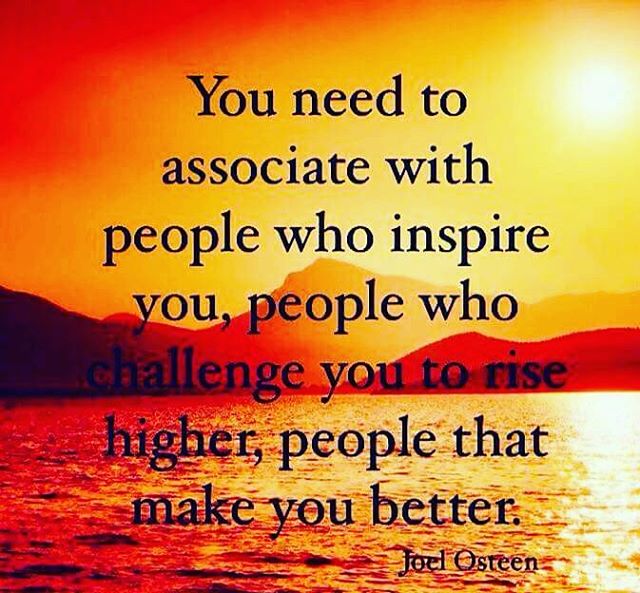The image is a square computer graphic intended for social media, featuring a highly saturated, sunset or sunrise scene over a tranquil lake flanked by hills and a mountain. The scene is bathed in vibrant hues of orange, yellow, and red. The water reflects these colors, with some subtle wave patterns, adding depth to the otherwise simplistic background. Dominating the upper portion of the image is a motivational quote in black text: "You need to associate with people who inspire you, people who challenge you to rise higher, people that make you better." This quote is attributed to Joel Osteen, whose name appears in the bottom right corner. The overall setting, devoid of any people or boats, keeps the focus on the uplifting message.